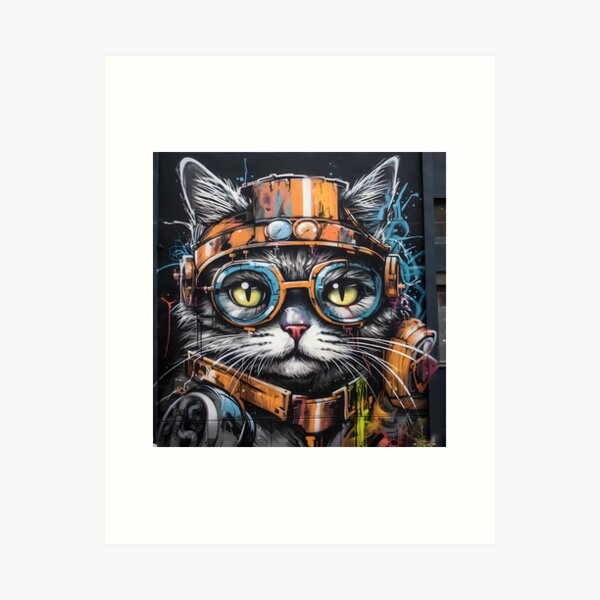This detailed image is a graphic illustration of a futuristic, cyberpunk-styled cat, prominently featured against a dark background with a mix of turquoise blue and red paint strokes. The cat, depicted in a black square within a white vertical rectangle, which is enclosed by a light gray boundary, is shown from the head down to a metallic neck guard. The gray and white cat, possibly with some black hairs, has large greenish-yellow eyes with vertical slits and a pink nose. It's wearing an elaborate steampunk helmet that appears metallic and slightly worn, featuring a band across the forehead with small colored circles and an orange rectangular piece between its ears. The helmet is complemented by matching orange-rimmed goggles with translucent blue lenses. Long white whiskers extend to the left and right of its face. Around its neck, the cat wears a complex metallic neck guard or belt with bolts and a clasp, resembling a piece of armor. This part continues to a small orange component on the right side, partially obscured by whiskers. The entire portrayal suggests a setting where the cat looks serious and ready, perhaps as a space worker or futuristic adventurer.